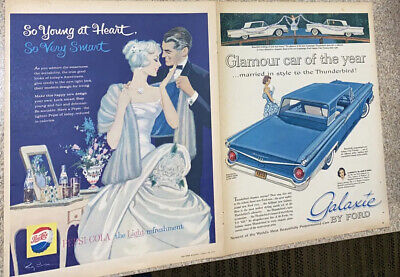The photograph depicts a vintage magazine, slightly yellowed with age, placed diagonally on a grey, speckled countertop. The magazine reveals a double-page spread, each side showcasing different advertisements. On the left-hand page, a cartoon illustration features a smartly dressed couple: the woman in an elaborate white ball gown and the man in a dark navy tuxedo with a bow tie. They appear to be on the brink of a kiss, with the woman tenderly holding the man's chin. Above them, white text on a navy blue backdrop states "So Young at Heart, So Very Sweet." Below them, there's a nightstand adorned with a mirror, various bottles, and small flowers, suggesting a getting-ready scene. A prominent Pepsi Cola logo and cap are also depicted.

On the right-hand page, a blue 1960s car, complete with long wings, red taillights, and chrome bumpers, is shown from the rear. The text "Glamour Car of the Year" appears at the top against a white background, alongside smaller illustrations of cars. At the bottom right, the word "Galaxy" is artistically rendered in blue, followed by the phrase "Buy Ford" in bubble-style black text. Additionally, a woman in a blue dress opening the car's left door adds to the vintage allure, emphasizing the advertisement's nod to nostalgic elegance and sophistication.